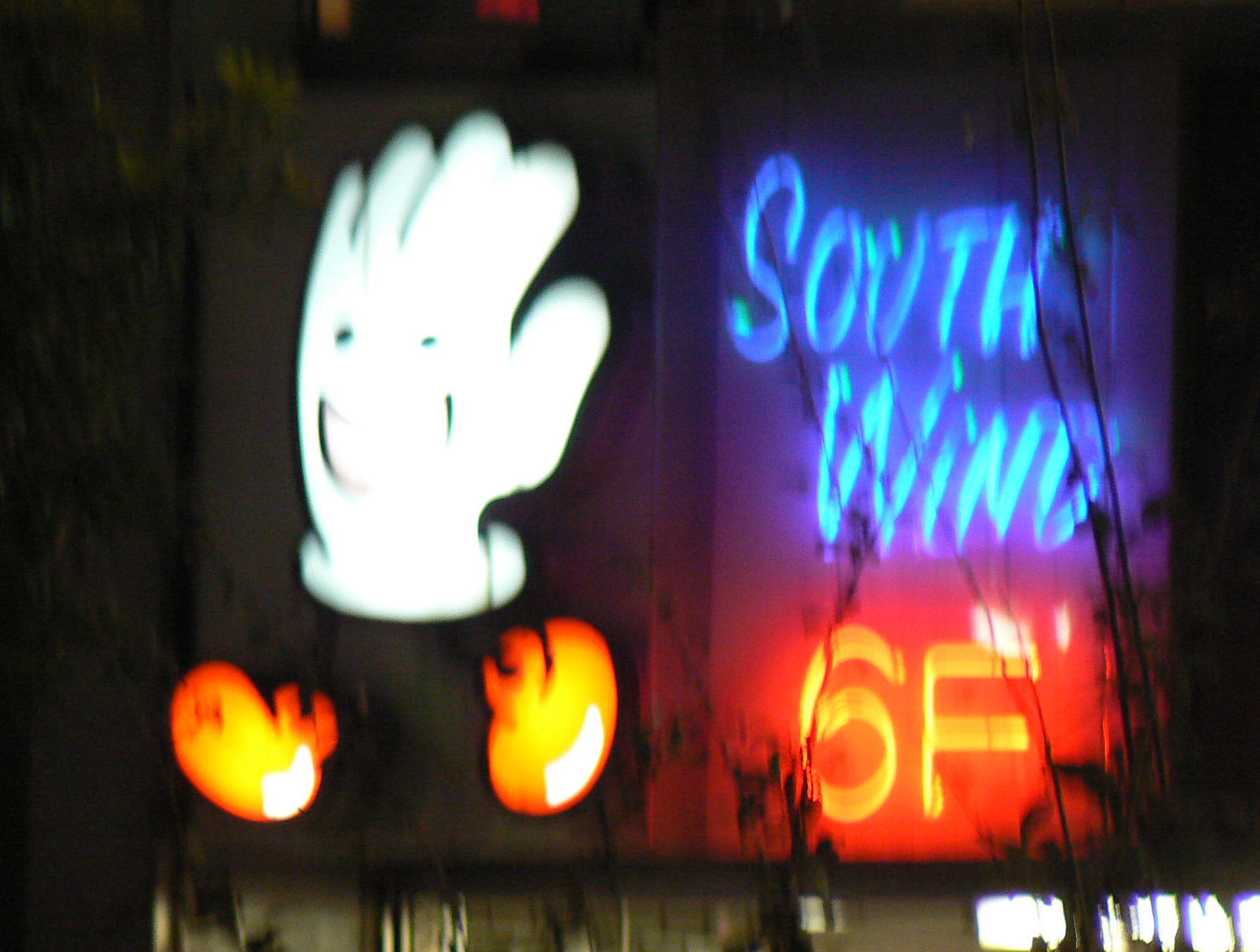An out-of-focus landscape-format photograph captures the blurred yet colorful neon signage of an establishment at night. The image, taken outdoors, features a dark backdrop with the faint silhouettes of branches on the right side. Prominently displayed on the left side of the frame is a whimsical neon mascot—a white glove with a smiling face and orange shoes, seemingly walking toward the left. On the right side of the sign, the name of the establishment is illuminated in striking blue neon letters that read "South Wind," beneath which the characters "6" and "F" are lit up in bright orange.